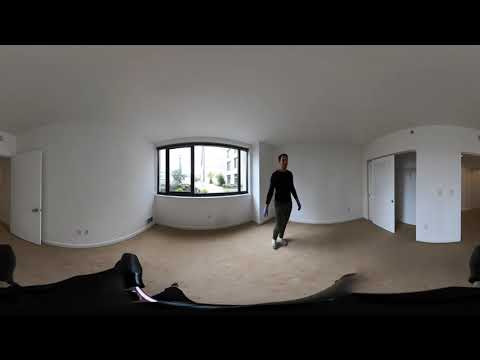This is a small, rectangular horizontal image depicting the interior of what appears to be an unfurnished living room taken with a special 360-degree lens, creating a convex, curved effect on the white walls and ceiling. The focal point is a man, likely Caucasian with short dark hair, standing on the brownish or beige floor, dressed in dark clothes including a black long-sleeve shirt or sweater, grayish pants, sneakers, and wearing surgical gloves—possibly indicating he is in the process of cleaning the space. To his left, there is a window framing an outside view of trees and some buildings, suggesting it is daytime. The window lacks blinds or curtains. Additionally, on the far left side, there's a door leading to another room and another door visible on the right, possibly to a closet. In the foreground, there appears to be a curved piece of furniture with cushions. Overall, the room gives an impression of being empty, possibly ready for sale or rent.